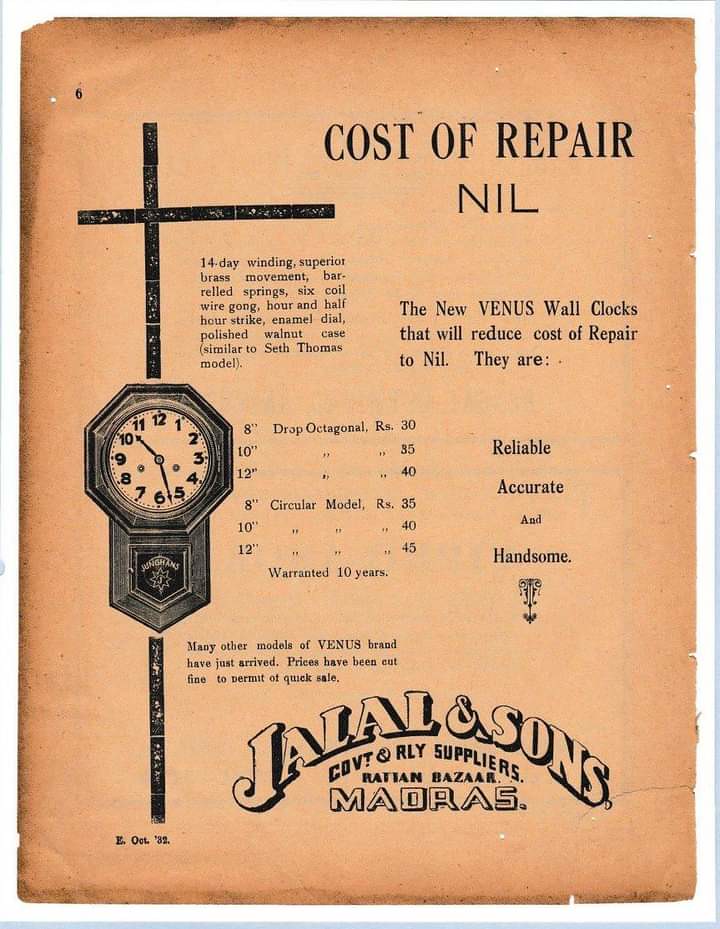This vintage 1932 advertisement, likely from India, showcases a well-worn but preserved vertical rectangular piece of orange-brown paper with a slightly torn upper left corner and small rips along the right and bottom edges, accompanied by overall wrinkles. The centerpiece of the left-hand side is a vertical black line that features a horizontally crossed top and an outline of a clock, displaying 10:28 with detailed descriptions including "14-day winding," "superior brass movement," "barreled springs," "6 coil wire gong," "hour and half-hour strike," "enamel dial," and "polished walnut case," similar to a Seth Thomas model. 

On the upper right side in bold black caps, the advertisement declares, "COST OF REPAIR, NIL." Below this, it promotes the new Venus wall clocks with the text: "The new Venus wall clocks that will reduce cost of repair to nil. They are reliable, accurate, and handsome." Each of these qualities is centered over a logo. The bottom of the page, curved centrally, reads "Jalal and Sons" in outlined block letters, followed by "GOVT. RLY suppliers" and "Ratan Bazar, Madras," suggesting the company's location and market. This historical artifact reflects the bygone era's craftsmanship and commercial aesthetics.